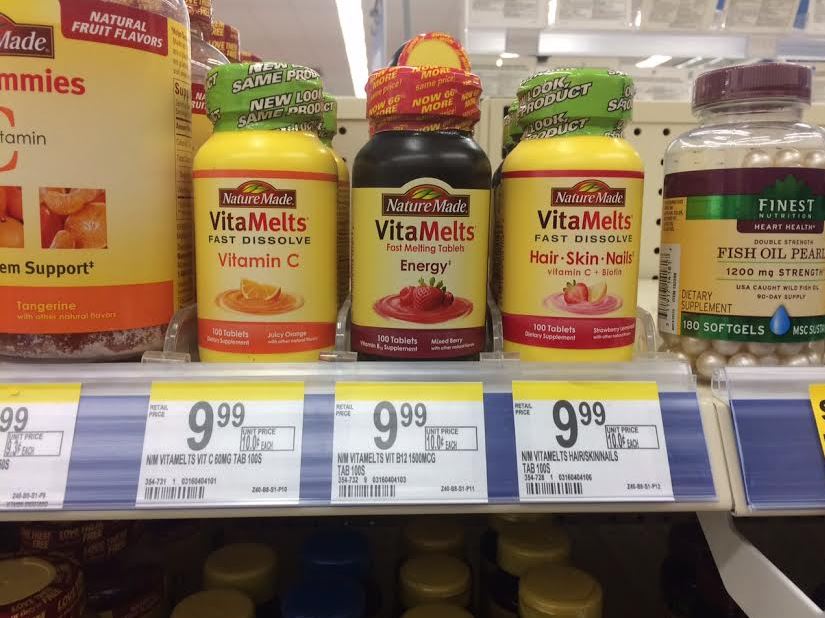The photograph captures a well-organized pharmacy aisle inside a grocery store with a focus on various vitamin bottles. Prominently featured are several Nature Made vitamin bottles and a single transparent bottle labeled "Finest Fish Oil Pearls." This transparent bottle, positioned to the right, contains smooth, shiny pearls that indeed resemble actual pearls, with their lustrous white appearance embodying an elegant look.

Adjacent to the Finest Fish Oil Pearls bottle are three medium-sized Nature Made vitamin bottles. The two outer bottles are a vivid yellow with green caps, while the bottle in the center stands out with a darker hue, possibly dark red or purple, and a distinctive red cap paired with a yellow label. Further to the left, a large bottle of Nature Made Vitamin C gummies can be seen, recognizable by its light yellow label and what appears to be a red cap. The detail and variety of bottles display a range of options available to shoppers seeking vitamins in this section of the store.